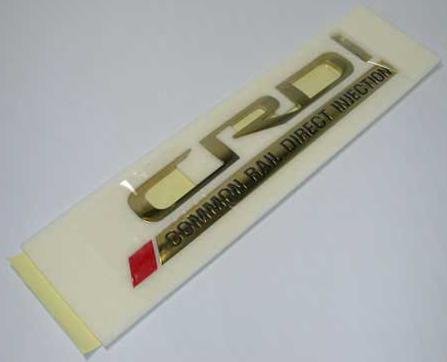The image showcases a long, rectangular badge, oriented at a diagonal angle from the bottom left to the upper right corner. The badge prominently features silver or gold-colored lettering on a white background, spelling "C.R.D.I." Below this, there is a raised, silver or golden bar with the text "Common Rail Direct Injection" engraved on it in smaller, dark lettering. To the left of this text bar is a small red chevron, or polygon. The badge itself is tilted at about a 45-degree angle, and appears to be lying on a thin, yellow piece of paper, possibly a post-it note, with a grayish-white background visible behind it. Some yellow appears to be showing through the "C" and "D" in the "C.R.D.I." logo.